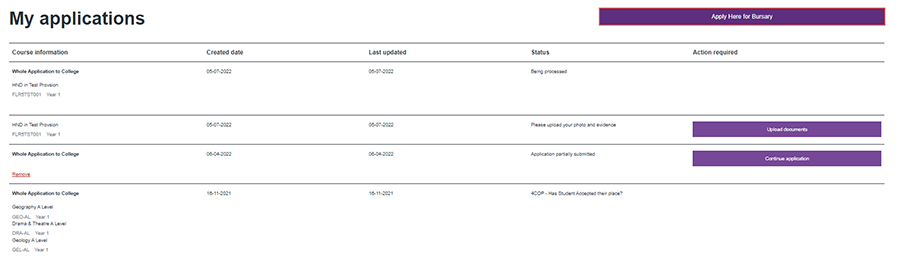This is a cropped screenshot of the "My Applications" section within a college application program. The header at the top left displays "My Applications" in bold black font against a clean white background. On the top right, a prominent purple button labeled "Apply Here" is visible—although the specific college name on the button is too small to read. This button is encased in a red, edited box to highlight that it is the call-to-action for initiating an application.

Below the header, a row of categories organizes the application details, including "Course Information," "Created Date," "Last Updated," "Status," and "Action Required." The first row under "Course Information" displays an application to a college, detailing the date it was created, the last updated date, and indicating its current status as "Processing." 

Below that, a second application entry shows its details, along with a status message reading "Paused until you pay," indicating that some step in the process is pending financial action.

The third row lists another application with a red line underneath to signify a new entry. Both the second and third applications have adjacent action boxes for further management.

Finally, there is an additional application entry at the bottom of the section, which has an error status.